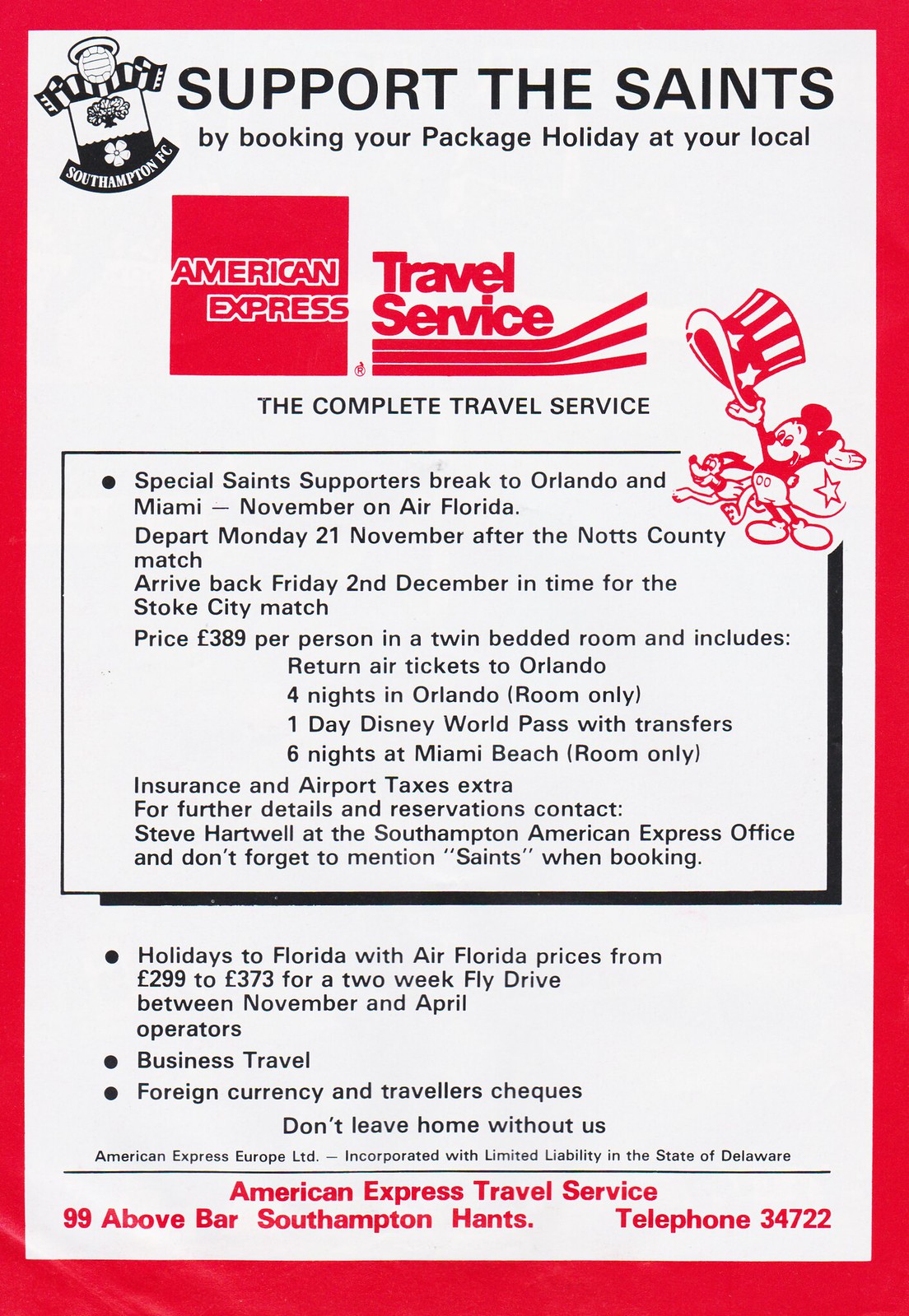The image is an advertisement with a white background and a thick red border surrounding the entire page. At the top, in large black capital letters, it reads "SUPPORT THE SAINTS." Just below this, a smaller print urges readers to "book your package holiday at your local American Express Travel Services."

In the top left corner, there is a logo that resembles a soccer ball, a scarf, or a poster, but it's not very clear. Further down, the page highlights a promotion with black text on a white background. This is a "special Saints supporter break to Orlando and Miami in November via Air Florida," departing Monday, November 21, after the Knotts County match and returning by December 2. Additional details and pricing information are provided in three bullet points.

Near the center of the page, there's a red square housing the American Express logo, accompanied by the text "Travel Service" with lines underneath, and below it, "The complete travel service" in black letters. In the bottom left corner, you find another instance of "American Express Travel Service," with the address "99 Above Bars, Southampton" and a telephone number "34722" listed underneath.

In the right corner of the flyer, there is an image of Mickey Mouse tipping his hat, accompanied by Pluto, signifying the Orlando destination package. The flyer is primarily an advertisement for Southampton FC (potentially indicated as "Saints"), with a call to support the team by using American Express Travel Services for booking holidays.